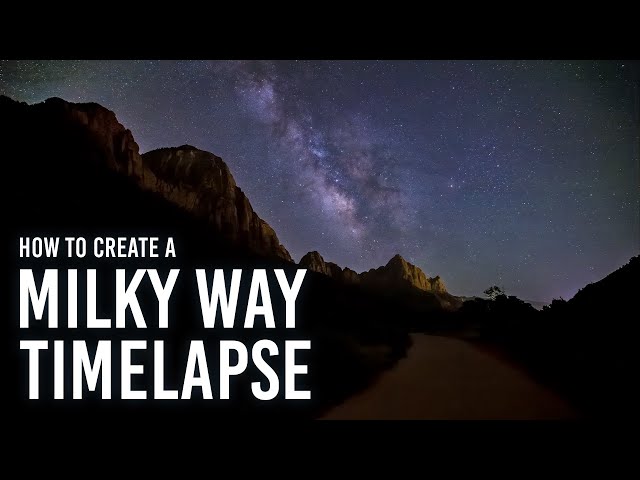This screen capture from a video tutorial titled "How to Create a Milky Way Timelapse" showcases a captivating night scene set in a canyon. The foreground features a dirt walking path, bordered on the right by tall, rocky mountains and on the left by tree-topped hills. Both the mountainous and hilly landscapes are silhouetted against the completely dark sky, which is adorned with countless illuminated stars, creating a vivid view of the Milky Way. The Milky Way's clarity dominates the upper half of the image. Notably, there are thick black borders at the top and bottom of the still, adding to the dramatic effect. Text on the lower left corner reads, in white lettering, "How to Create a Milky Way Timelapse," indicating that this image serves as a YouTube thumbnail for the tutorial. Occasional light pollution slightly illuminates parts of the mountains, adding depth to the scene.